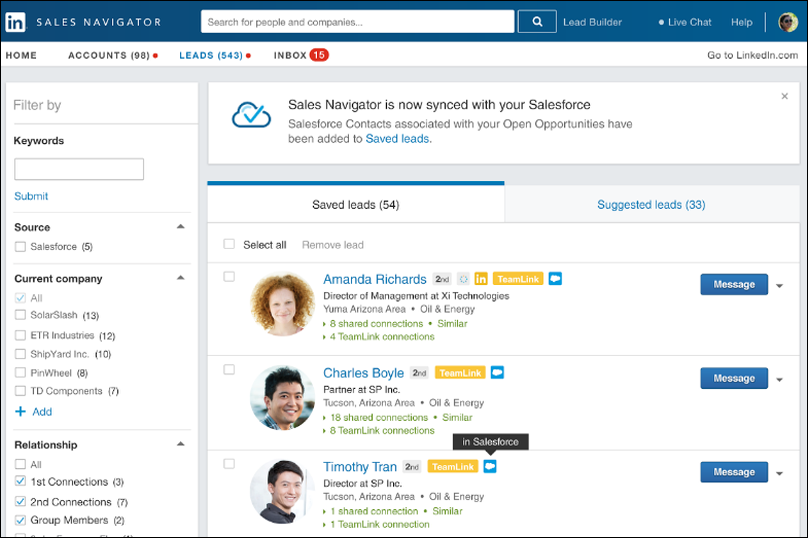Here’s a cleaned-up and detailed caption of the described LinkedIn page:

"The top section of the LinkedIn Sales Navigator webpage is predominantly blue. At the top left, there is a white LinkedIn logo displayed within a blue box alongside the text 'Sales Navigator' in white. Below this, there's a white search bar with gray text that reads 'Search for People and Companies,' accompanied by a magnifying glass icon. Adjacent to the search bar, there's a blue button with a white border labeled 'Lead Builder.' Additionally, 'Live Chat' and 'Help' links are visible nearby.

The navigation menu below includes several tabs, mostly in black, except for the third tab, highlighted in blue, indicating the current section. The tabs read 'Home,' 'Account 298' with a red notification circle, 'Leads (543)' also with a red notification circle, and 'Inbox (15)' with a red background.

Further down, there's a filtering section that starts with 'Filter by' followed by a white input box for 'Keywords.' A blue 'Submit' button and selections for 'Source' which includes 'Salesforce (5),' 'Current Company' with multiple options like 'Solar/ETR, Shipyard Inc., Pinwheel, TD Components,' and in blue, 'Add.'

Under 'Relationship,' different connection options are listed, such as 'First Connection,' 'Second Connection,' and 'Group Members.' 

Below these filters, options to 'Save Leads' and 'Select or Remove Leads' are available. Specific contacts are listed such as 'Amanda Richards,' 'Charles Boyd,' and 'Timothy Tran,' all highlighted in blue, suggesting clickable links. To the right of each name, there is a blue button labeled 'Message' in white font, indicating the option to send a direct message to these individuals."

This detailed caption provides a clear visual and functional overview of the LinkedIn Sales Navigator interface as described.